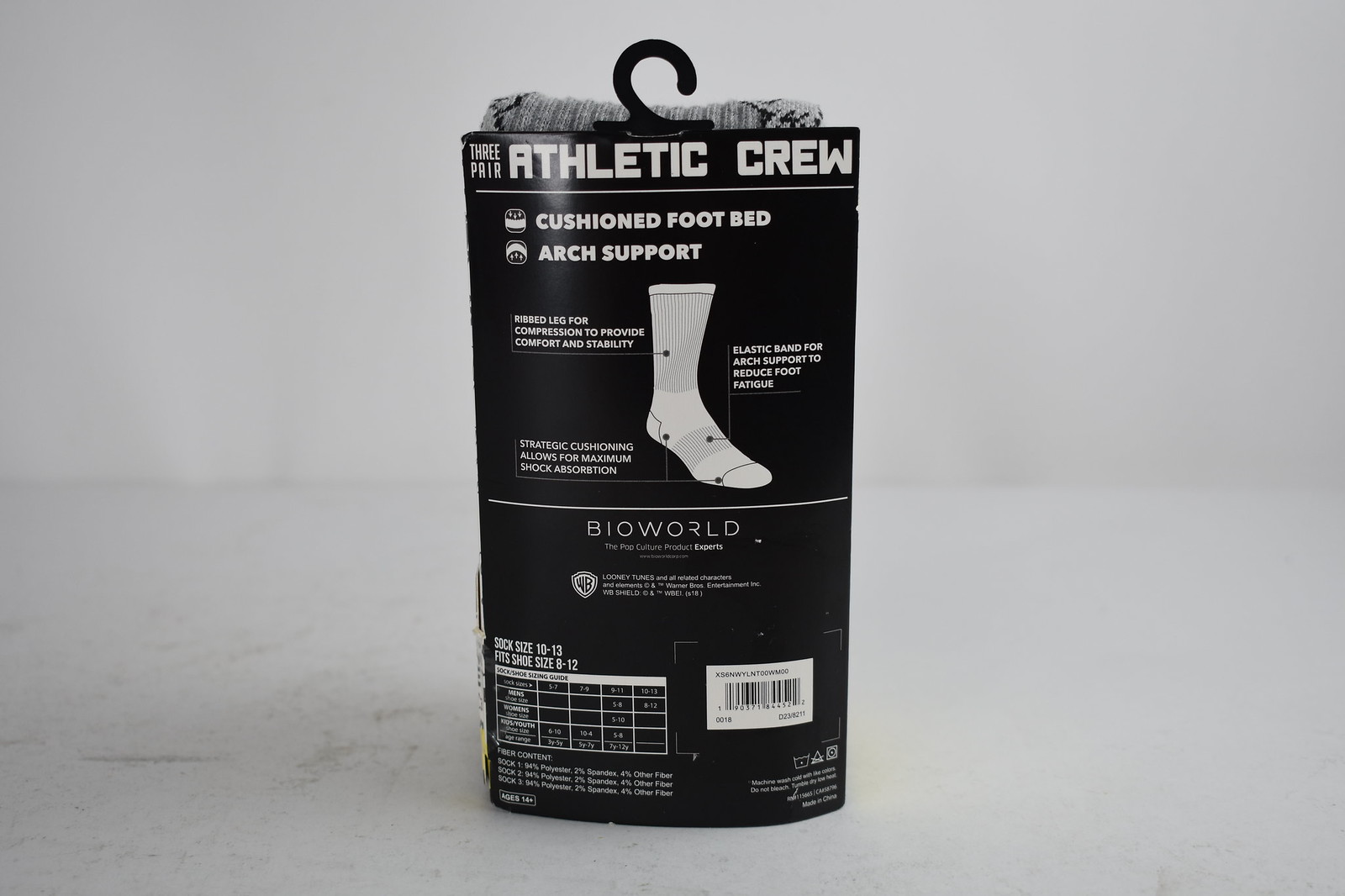The image depicts the back of a black packaged set of three athletic crew socks, displayed on a slightly dirty white tabletop with gray marks on the left side. The prominently visible black hang tab at the top of the package is designed for easy display. The package reads "Three Pair Athletic Crew" in white font at the top. Below that, there are highlighted features: "Cushioned Footbed," "Arch Support," and a technical illustration of a white crew sock pointing to features like "Ribbed Leg for Compression," "Strategic Cushioning for Maximum Shock Absorption," and "Elastic Band for Arch Support to Reduce Foot Fatigue." The bottom section showcases the BioWorld logo, known for pop culture products, along with the Looney Tunes branding and the Warner Brothers (WB) logo, specifying "Looney Tunes and all related characters and elements © Warner Brothers Entertainment Inc." A sock size guide indicating "Size 10-13" (for shoe sizes 8-12) is shown on the lower left, while a barcode and additional details are present on the right. The top of the package reveals a glimpse of the gray socks inside. The overall lighting is good, providing clear details of the packaging design and text.